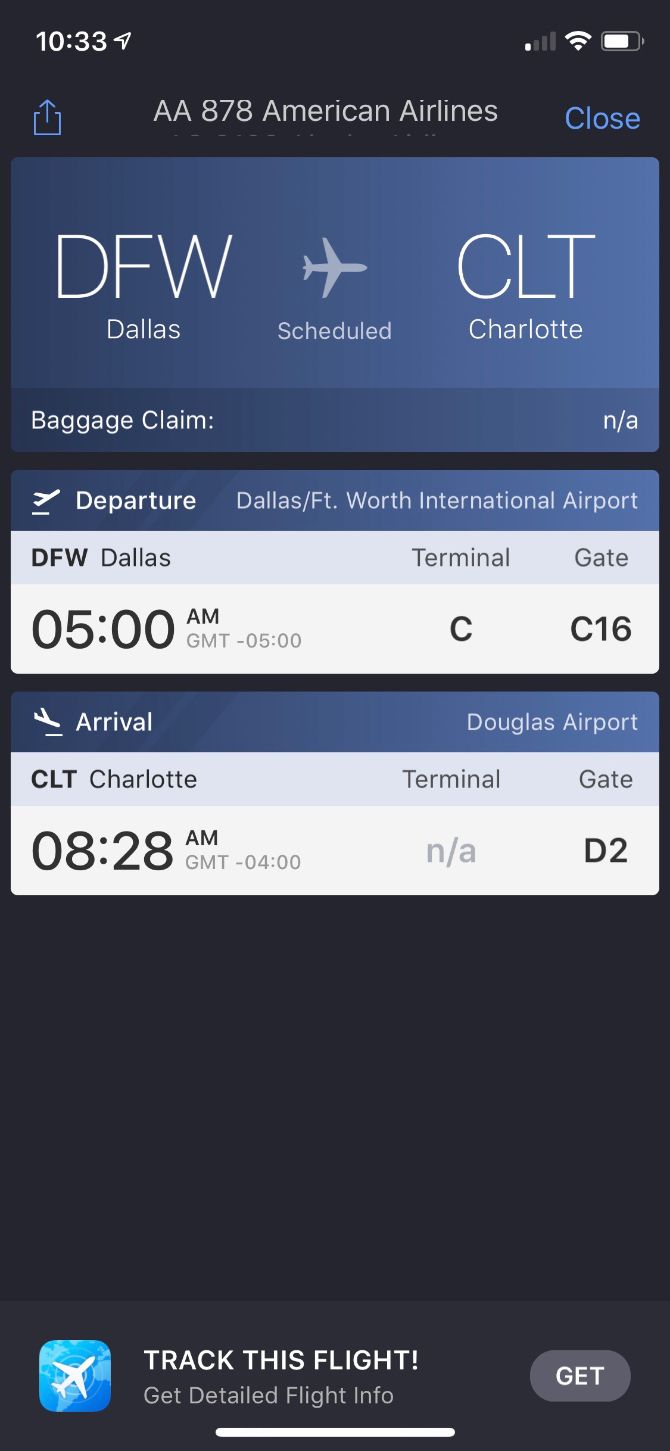Screenshot of a cell phone screen displaying flight information. The top section features a black status bar. On the left, it shows the time 10:33 in white text. On the right, icons including a GPS symbol, a single cell service bar, a fully connected Wi-Fi signal, and a battery indicator at 75% are visible. Just below, a blue box with an upward arrow appears, meaning unknown.

The main body of the screen contains detailed flight information in various shades and colors. The top left displays "AA 878" in gray text, indicating the American Airlines flight number. Adjacent to it, "on time" is written in blue text on a blue background. Below it, "Origin" is indicated as "Dallas/Fort Worth International," abbreviated as "DFW," in black text on a gray background.

Further down, a blue plane icon is shown next to the label "Scheduled." The departure information follows: "Dallas Fort Worth International" in gray text, "Terminal C" in smaller black text, and "Gate C-16" all hinting at the departure location specifics. The expected departure time is 5:00 a.m.

Arrival details are listed next: "Charlotte" (abbreviated "CLT") in white text on a blue background, "Baggage Claim" location noted but not specified, and "Arrival at 8:28 a.m." in smaller black text. The terminal and gate details for arrival are stated as "unknown" and "D2" respectively.

At the bottom of the screen is a blue square with a white airplane icon, labeled "Track this flight" in white text, and below in smaller gray text, it reads "Get detailed flight info." To the right, a gray circular button with the word "Get" in white text is visible. At the very bottom center is a light bar, possibly indicating an interactive element or focal point.